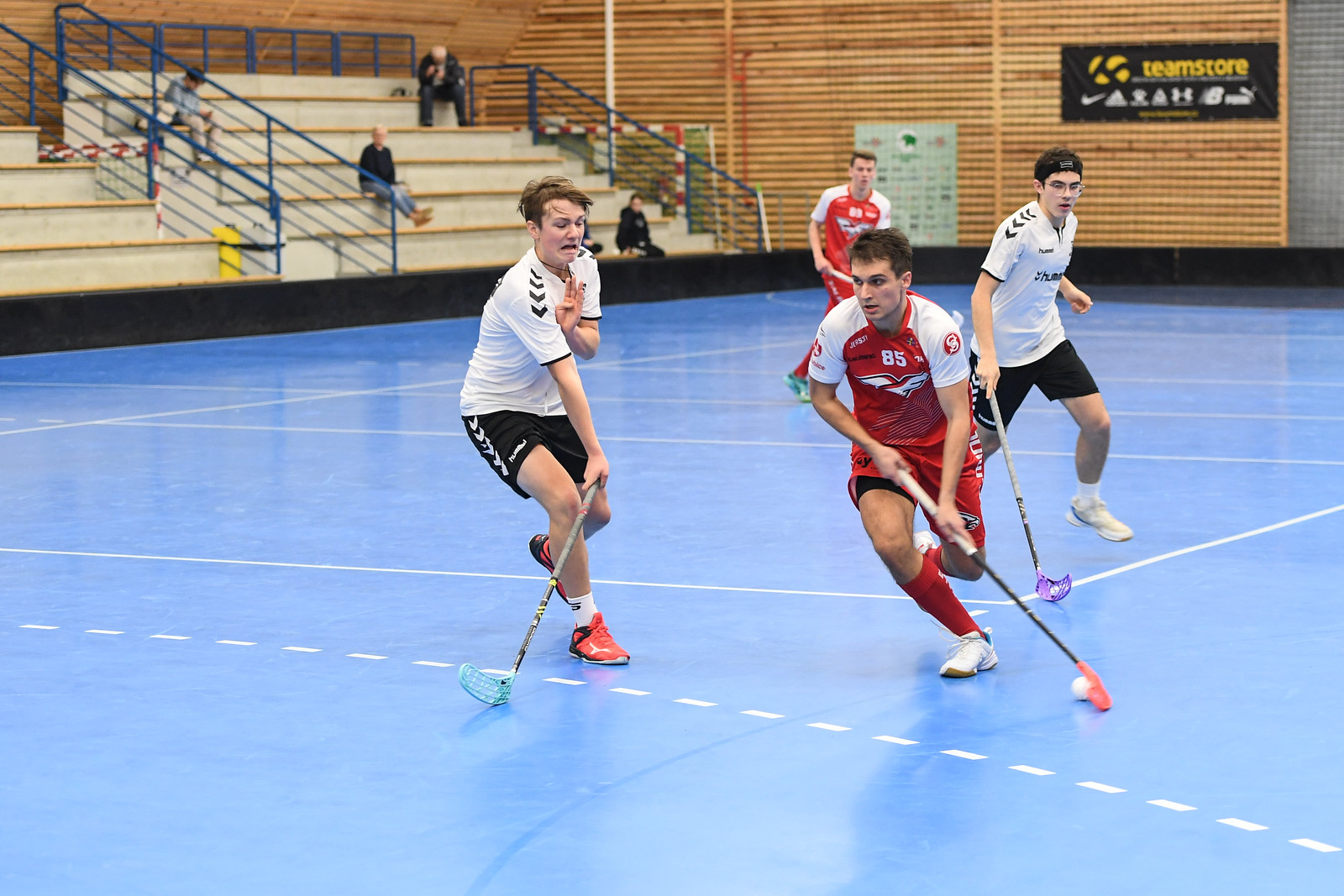The indoor photo captures an intense moment during a game of indoor hockey on a sky-blue gym floor. Four men are actively engaged in the game, divided into two teams. One team wears red jerseys with matching red shorts and socks, while the opposing team sports white jerseys with black shorts. The man in the red jersey is currently in possession of the ball, with a teammate in the background. Two players from the opposing team are seen rapidly approaching him, poised defensively with their hockey sticks. The scene is set within a gym with brick walls and a few wooden and grayish accents. To the left, a sparsely populated set of bleachers holds about four spectators, each sitting a distance apart, observing the action. A sign prominently displaying "Team Store" adds to the indoor sports atmosphere.